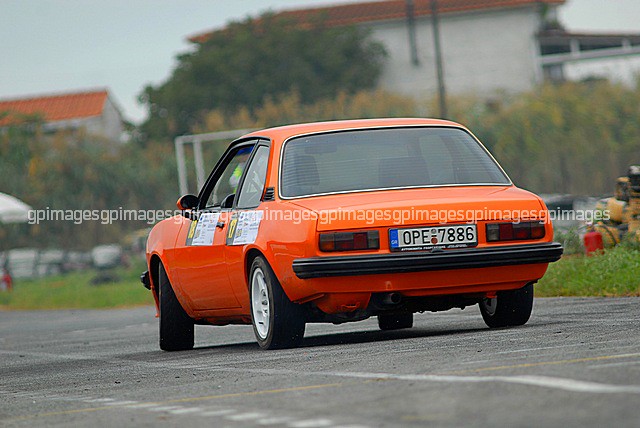In this detailed landscape photograph, taken outdoors during daytime, the primary focus is an older, possibly late 70s or early 80s, burnt orange two-door sedan with a fresh custom paint job featuring slight yellow accents. This car, which appears to be restored, is seen from a rear angle as it drives away on a regular asphalt road resembling a racetrack. The asphalt, occupying the bottom portion of the image, features a white line extending from the lower right to the upper left. The car, positioned directly in the center of the image, has a black bumper, white rims, a license plate reading OPE7886, and stickers on the driver's (left) side, including a green and white banner displaying yellow numbers that are partially visible. Surrounding the road is a green field with some scattered objects, a row of trees, and blurry house rooftops in the upper left background, all under a gray sky. A repeating "GP Images" watermark in various shades of gray, white, yellow, orange, blue, and red spans horizontally across the center of the image.